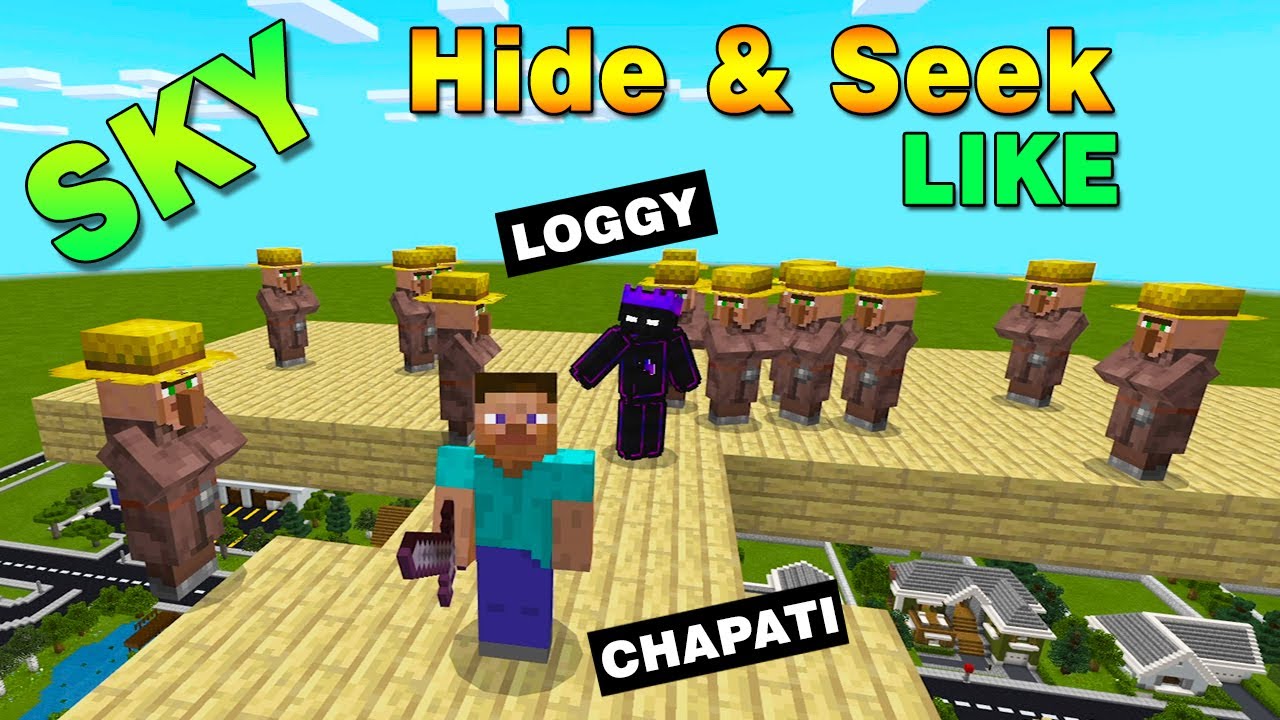This screenshot from a pixelated video game, likely Minecraft, captures a dynamic scene atop a yellow platform with a cityscape below. At the center, a character in a blue shirt and blue pants, wielding a sword, gazes directly at the camera. Surrounding them are figures dressed in brown outfits with yellow farmer hats, possibly signifying workers or an army. A notable character in the middle, clad in black and adorned with a purple crown, stands out as a potential leader. Text elements enhance the scene: at the top, "Sky Hide-and-Seek" is prominently displayed, while black labels with white writing identify characters— "Loggy" next to the person in black and "Chapati" beside the one in blue.